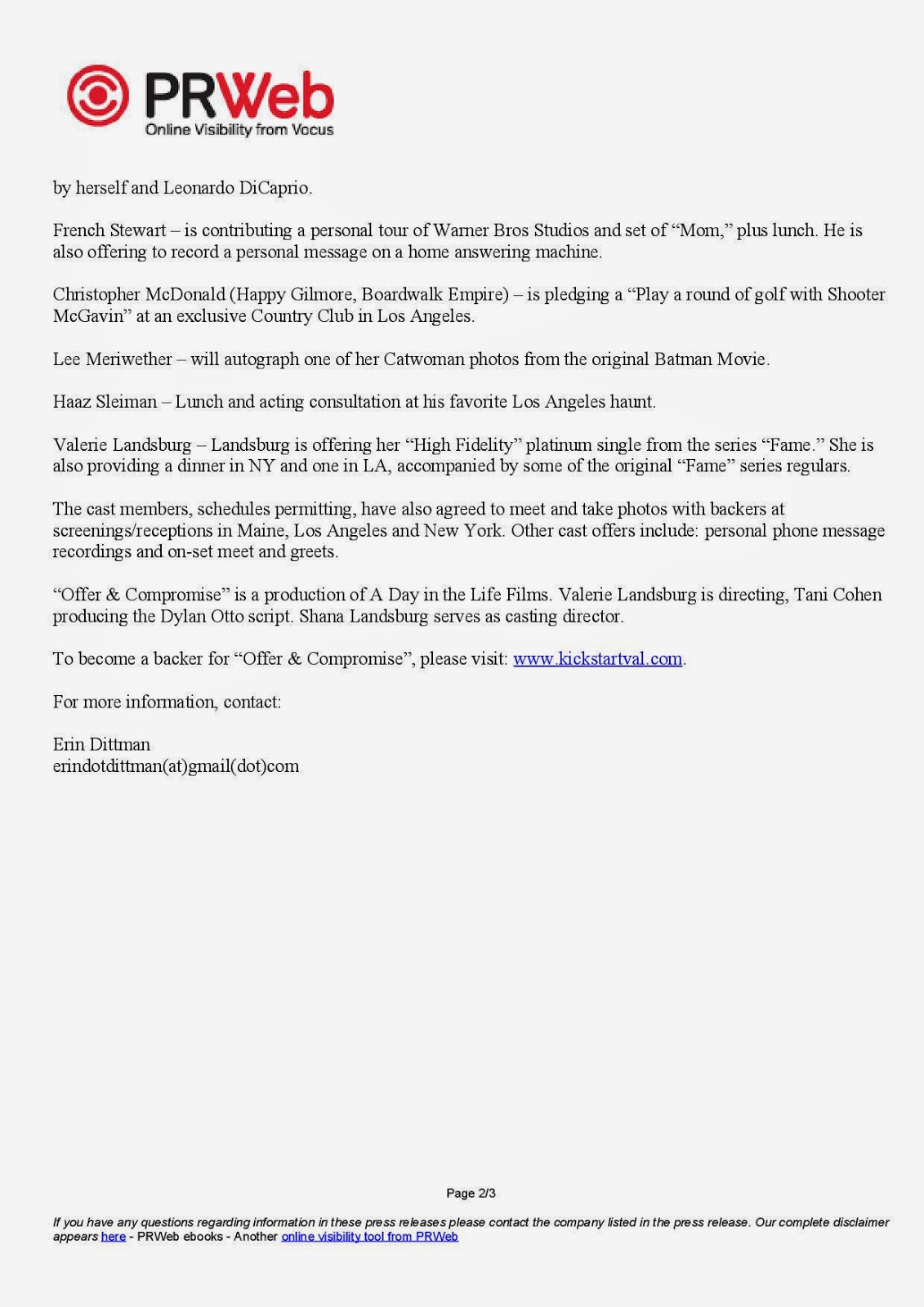Screenshot of a Press Release Page:

In the top left corner, a red circle with a dot in the middle indicates the source 'PR Web,' with the tagline 'Online Visibility from Vocus' beneath it. This is the second page of a three-page document, as noted at the bottom of the page.

Continuing from the previous page, the press release details several events and contributions involving notable personalities:

- **Herself and Leonardo DiCaprio:** French Stewart offers a personal tour of Warner Bros. Studios and the set of "Mom," complete with lunch. Additionally, he will record a personal message for a home answering machine.
- **Christopher McDonald (Happy Gilmore, Boardwalk Empire):** Pledges a round of golf with his iconic character, Shooter McGavin, at an exclusive country club in Los Angeles.
- **Leigh Merriweather:** Autographs one of her Catwoman photos from the original Batman movie, and offers lunch and an acting consultation at his favorite Los Angeles spot.
- **Valerie Landsberg:** Offers her high fidelity platinum single from the series "Fame," along with dinner in New York or Los Angeles, accompanied by some of the original Fame series regulars, schedules permitting.

Additionally, cast members have agreed to meet and take photos with backers at screenings and receptions in Maine, Los Angeles, and New York, subject to their availability. Other offers from the cast include phone message recordings and on-set meet-and-greets.

For more information, contact Erin Dittman at erin.dittman@gmail.com.